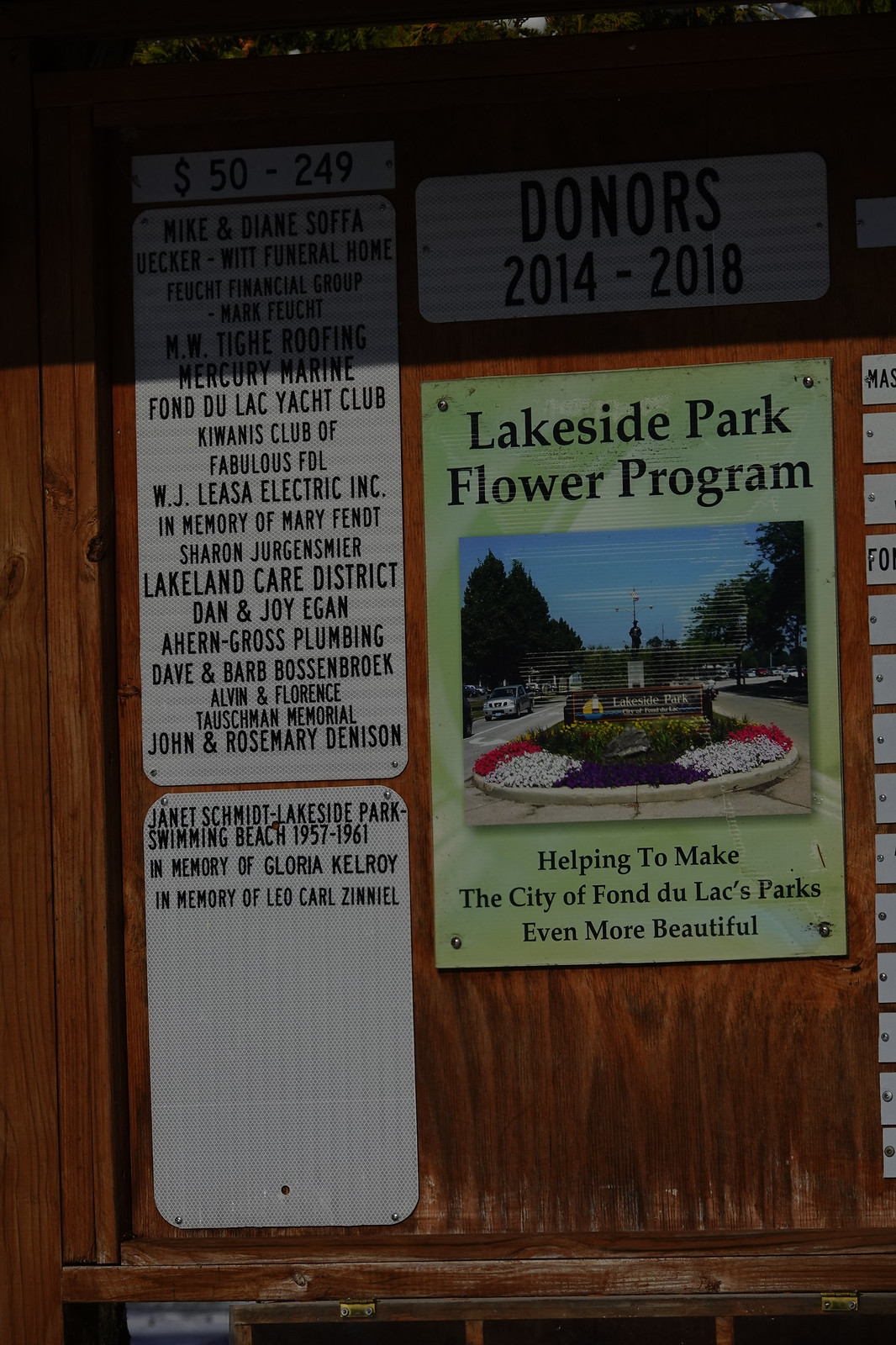The image is of an outdoor wooden billboard covered with various signs and a central color poster. The primary poster, with a green background, is titled "Lakeside Park Flower Program" and features a picture depicting an outdoor scene with a circular arrangement of red, white, and purple flowers. To the left of this floral display, there is additional text detailing the sponsors of the program. The image also showcases a fountain without water, surrounded by rocks and flowers, with trees and a road visible in the background. Above the central poster, a sign reads "Donors 2014 to 2018," and to its left, a smaller white sign lists names of donors who contributed between $50 to $249, including several "in memoriam" mentions. At the bottom of the main poster, the text states, "Helping to make the city of Fond du Lac's parks even more beautiful." The brown wooden board holds this green poster along with other white signs, creating an informative display for the Lakeside Park Flower Program.